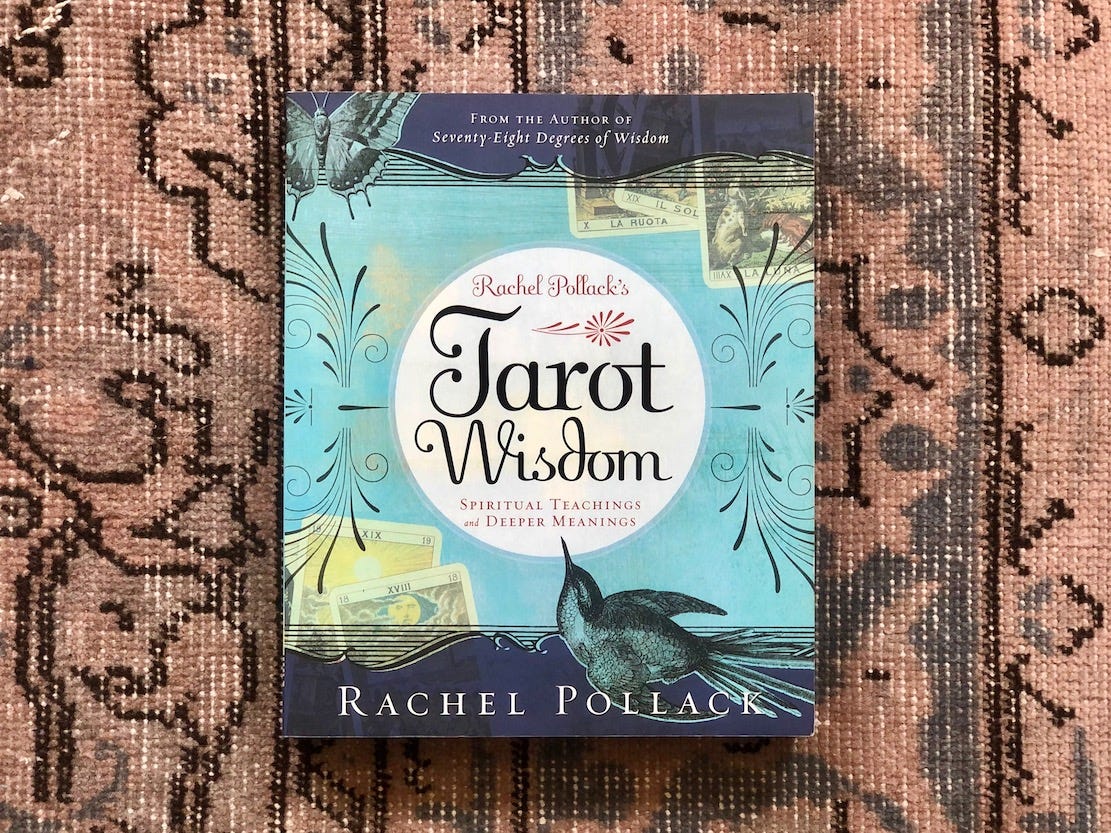The image is a close-up, horizontal photograph of a book titled "Rachel Pollack's Tarot Wisdom: Spiritual Teachings and Deeper Meanings." The book is lying on an old, threadbare, orange rug with black designs and visible white threads showing through. The book cover features a large white circle at the center with the title inside it, set against a blue background that darkens at the top and bottom. Above the title, it says “From the author of 78 Degrees of Wisdom.” A bird, possibly a hummingbird, is depicted on the right side of the cover, its beak reaching into the white circle. Rachel Pollack's name is prominently displayed twice, at the top and bottom of the cover, and next to the book, a few tarot cards can be seen scattered on the rug.